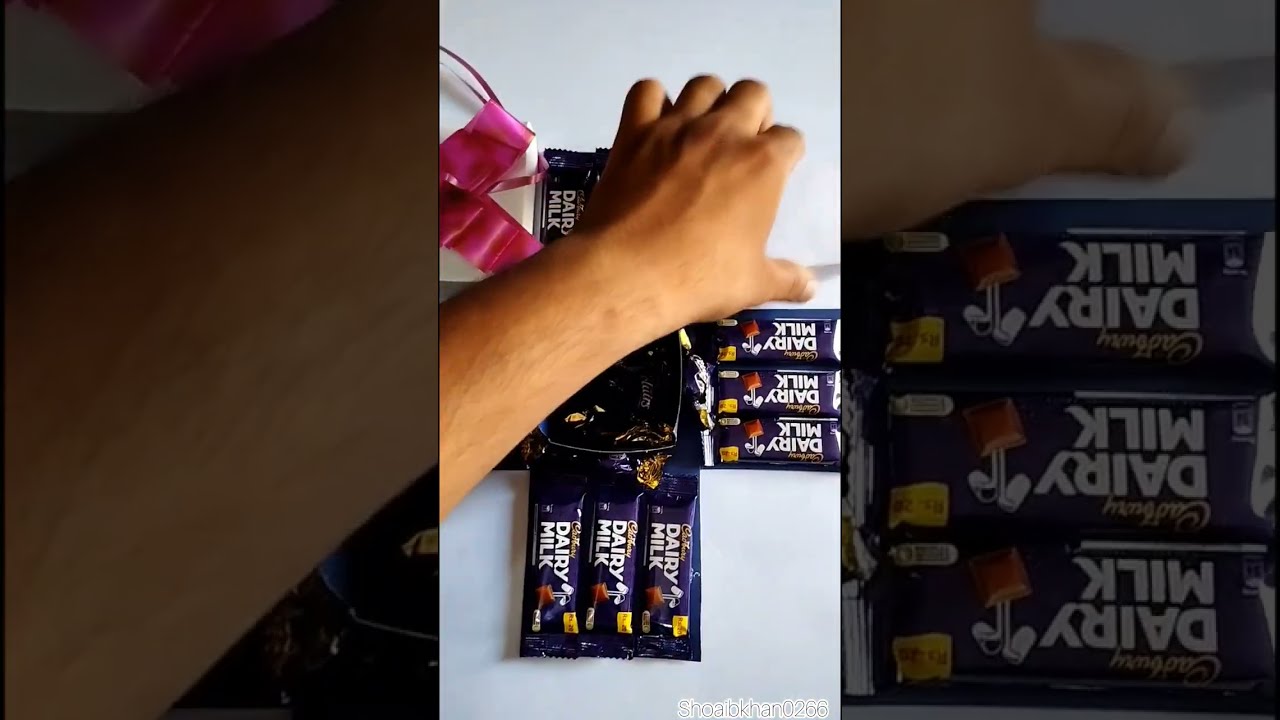In the photograph, a hand is reaching over an arrangement of Cadbury Dairy Milk chocolate bars, each wrapped in a distinctive navy blue wrapper with "Dairy Milk" printed in white letters. The candy bars, adorned with an image of chocolate and a small white plant, are meticulously placed to form an 'X' or cross pattern, with three bars at each point. The setup appears to be on a table, possibly suggesting a display or unboxing event. Adjacent to the bars, a white box tied with a pink ribbon adds an element of gift-giving to the scene. The periphery of the image features darker close-up sections: one side magnifying the chocolate bars and the other showcasing a portion of a forearm. Notably, the bottom right corner of the image displays the username "Shoaibkhan0266," hinting that this could be a promotional or sponsored content from a user-generated video.